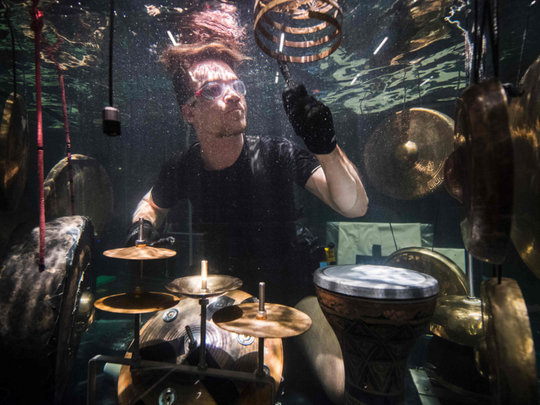The photograph captures a young man underneath the water, playing a makeshift drum set. He has short brown hair, is wearing clear goggles, a black shirt, and black gloves. Positioned at the very center, he appears to be either sitting or crouching. Surrounding him are various musical instruments: a gong behind him, multiple cymbals primarily in the center, a snare drum, and a bongo located near his right leg. Above him, there are floating devices and swirling objects, adding to the underwater ambiance. Additionally, red metal pipes or frames are noticeable to the side, along with a dangling microphone, which could be a special type designed for underwater use. The upper part of the image reveals water ripples and bubbles, indicating that this entire scene is just below the water's surface.